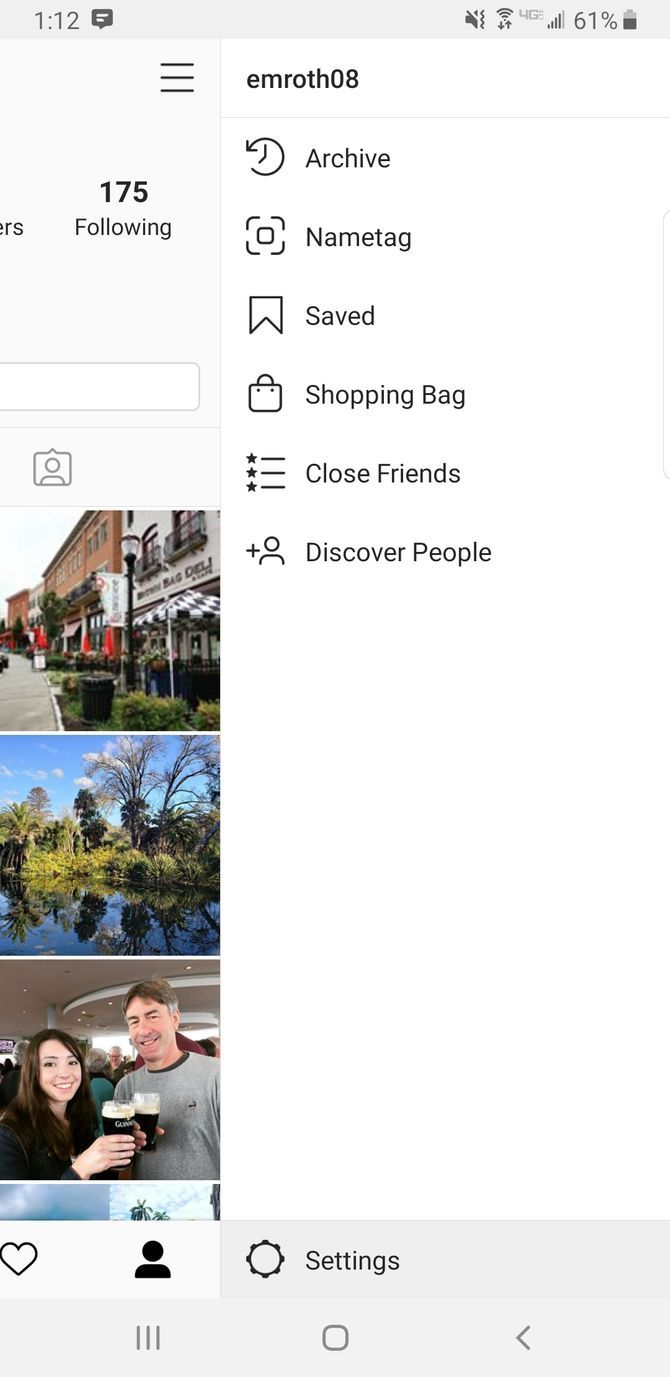The image is a detailed screenshot of an Instagram profile interface. At the very top of the screen, the time is displayed as 1:12. In the top corners, various symbols are visible: on the left, a back arrow indicating a navigation option, and on the right, icons showing a 61% battery level, 4G network connection, and that the sound is turned off. The profile handle "EMROTH08" is prominently displayed, with options for "Archive," "Name Tag," "Saved," "Shopping Bag," "Close Friends," and "Discover People" listed underneath, in that order, moving downward. 

At the very bottom of the screen, there's a "Settings" option. On the left side of the screen, the profile summary indicates that the user is following 175 people. Additionally, three thumbnail images are displayed: the first shows a bustling shopping center, the second depicts a serene river scene with surrounding plants, and the third captures a moment between a young woman and an older man clinking their Guinness cups together in a celebratory toast.